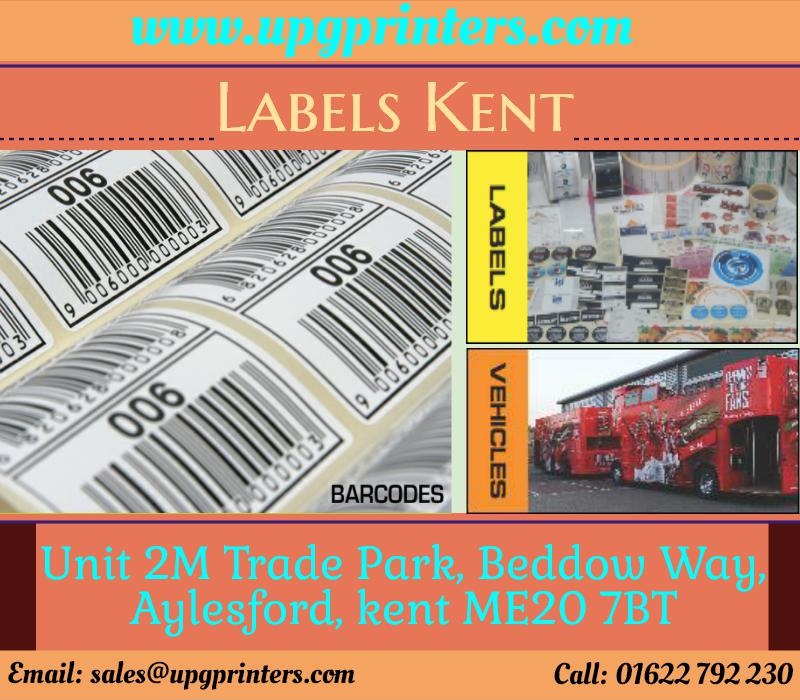The image appears to be an advertisement, likely for Labels Kent, displayed either in a magazine or as a poster. At the very top, there's an orange background featuring blue text that reads "www.upgprinters.com." Below this, in a more prominent orange font with yellow letters, it states "Labels Kent." The majority of the left side of the image showcases a variety of labels, including a label with the number "900" and a barcode. The right side of the advertisement exhibits labels of different shapes, colors, and sizes. Below these label images, there is a section highlighting vehicles, including a prominent reddish commercial vehicle. Further down, the address "Unit 2M, Trade Park, Beddow Way, Aylesford, Kent, ME20 7BT" is provided in an orange font with greenish letters. At the very bottom, the contact details are listed, including the email address "sales@upgprinters.com" and the phone number "01622 792230." The color scheme of the advertisement includes a diverse palette, featuring hues such as orange, light blue, dark orange, black, tan, white, yellow, red, blue, and purple. The structured layout of the images and information suggests this is an advertisement for a company specializing in the production of labels and promotional materials for vehicles.